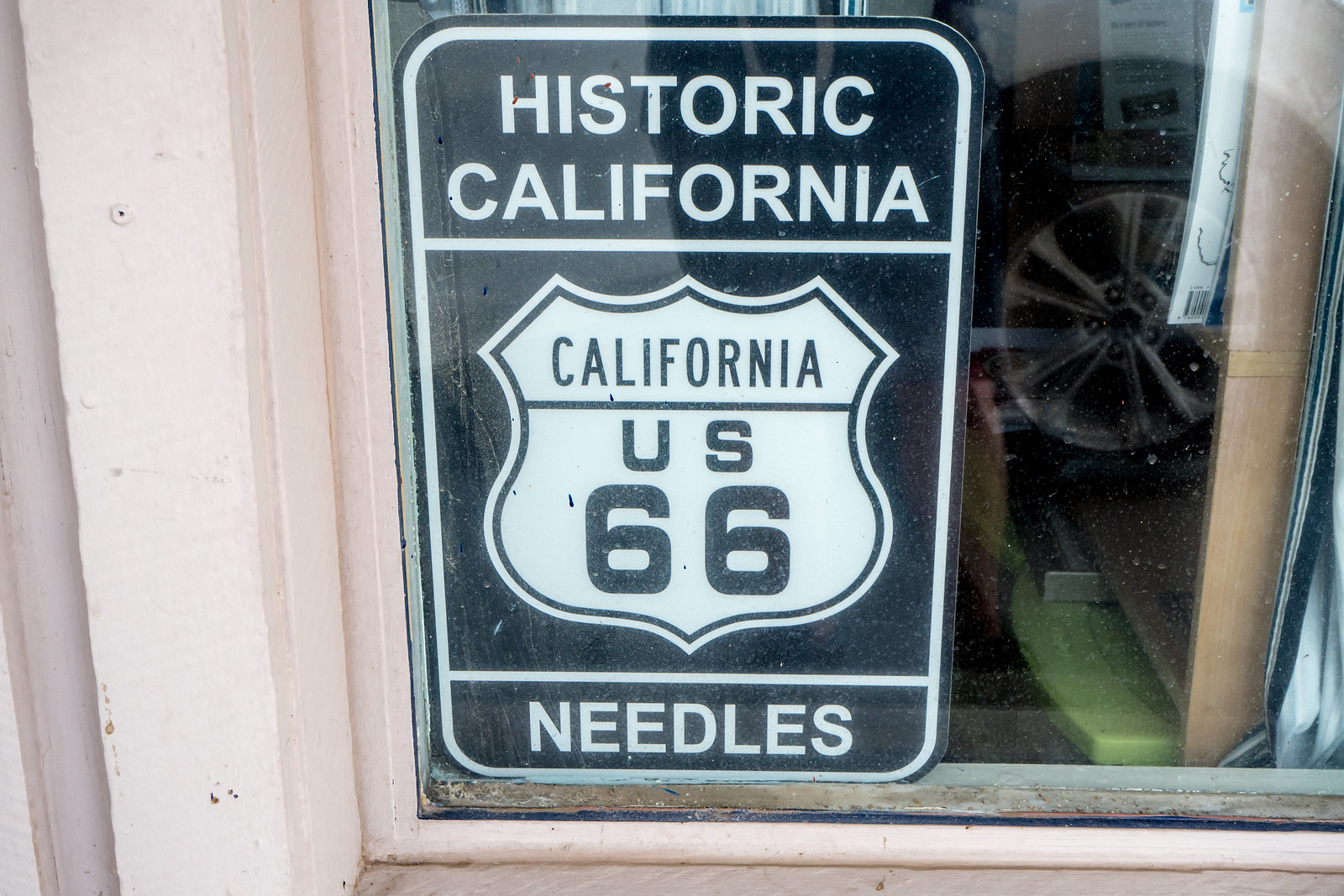The image depicts the front portion of a building, possibly a house or shop, with a prominently displayed black sign with white text in a window. The window has a light pink border, matching the exterior walls of the wooden building. The sign reads "Historic California" at the top, followed by a white line separator beneath which lies a Route 66 shield. The shield is labeled "California U.S. 66," and at the bottom of the sign, the word "NEEDLES" is displayed in all caps, separated by another white line.

In the reflection of the right side of the window, a tire from a vehicle is visible, indicating the presence of a car or vehicle parked across the street. Inside the building, behind the window, there appears to be a somewhat cluttered room with a ladder resting on a green counter, which has a wooden side extending up to the top right corner of the image. The overall scene suggests that the photograph was taken during the day, potentially on an overcast day, adding to the historic ambiance of the setting.